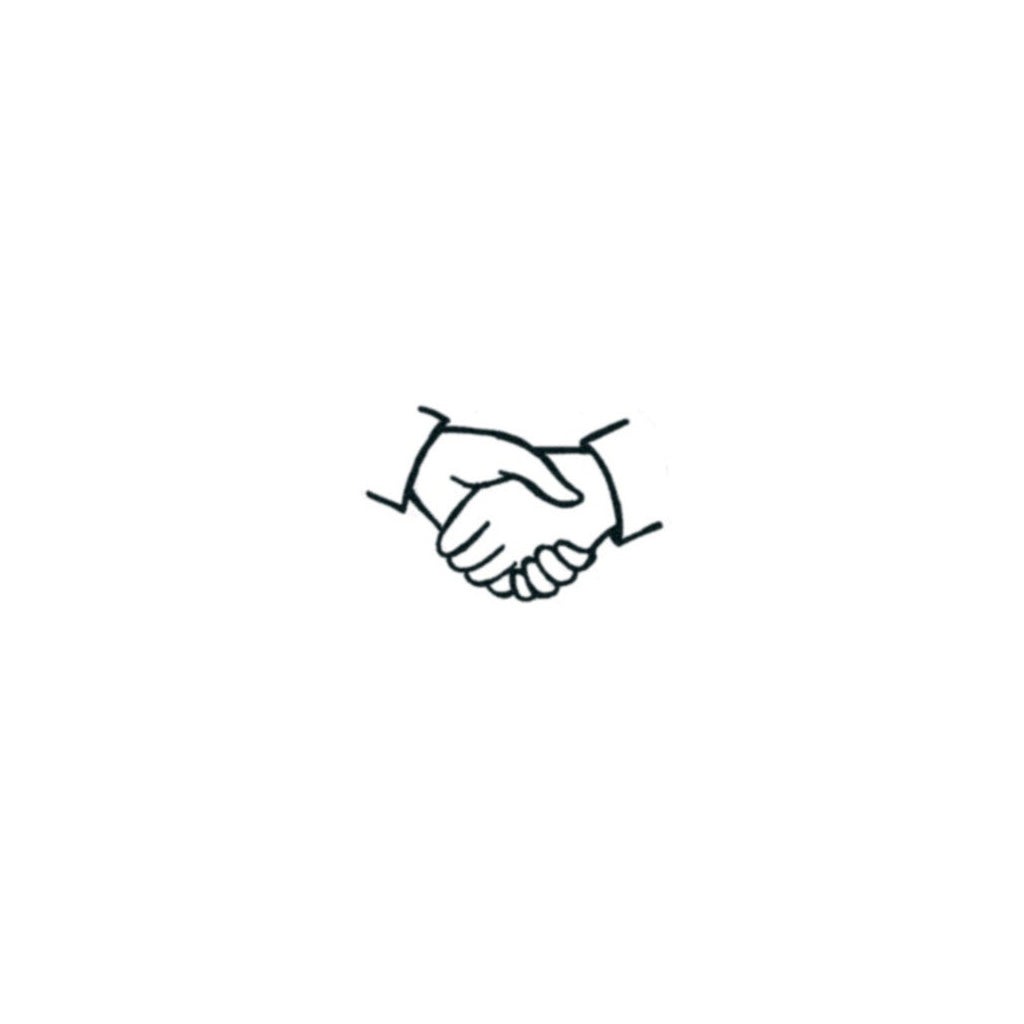The image is a simple, black-and-white digital drawing of two hands shaking, with a distinctively minimalist style. Both hands are clad in long sleeves, visible only at the wrists. The illustration is rendered in black lining with a stark white background, suggesting it could potentially serve as a logo or emblem. Notably, the drawing might have been created with a single continuous line, reflecting its seamless and clean design. The hands are oriented in such a manner that one can see the back of one hand and the palm of the other, with discernible fingers—three on one hand and four on the other. An intriguing detail is that both hands appear to be left hands, adding a unique element to the otherwise straightforward depiction. The overall aesthetic bears a resemblance to logos from insurance companies like State Farm or Allstate, highlighting its appropriateness for branding or symbolic purposes.